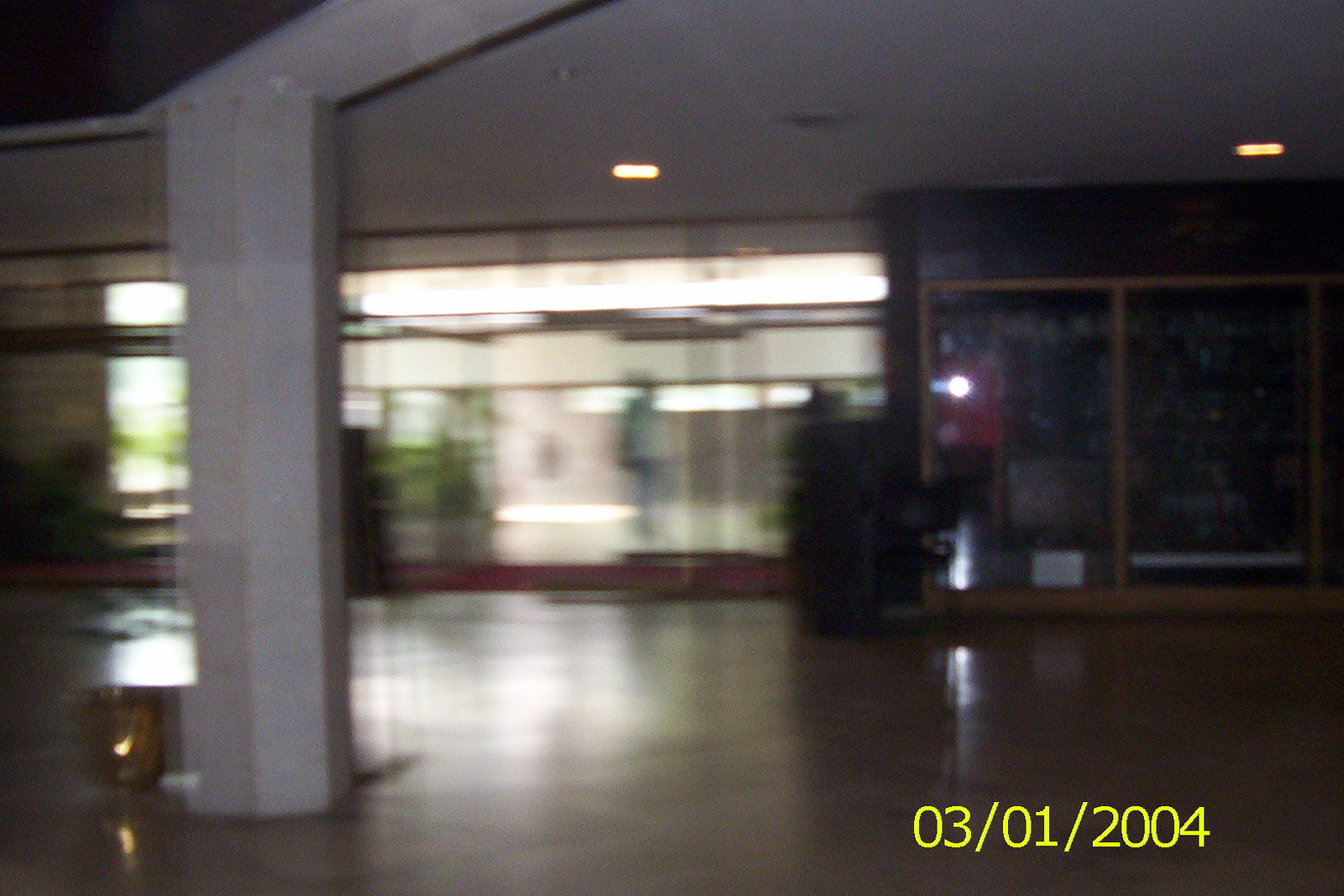A blurred, motion-captured photograph taken inside a dimly lit building. On the left side, a concrete pole prominently displays the date "03-01-2004," potentially indicating either March 1st or January 3rd, depending on regional formatting. Sparse ceiling lights attempt to pierce the darkness but fail to fully illuminate the space. Towards the back, doors or windows are visible, flooding the rear of the image with light, in stark contrast to the shadowed foreground.